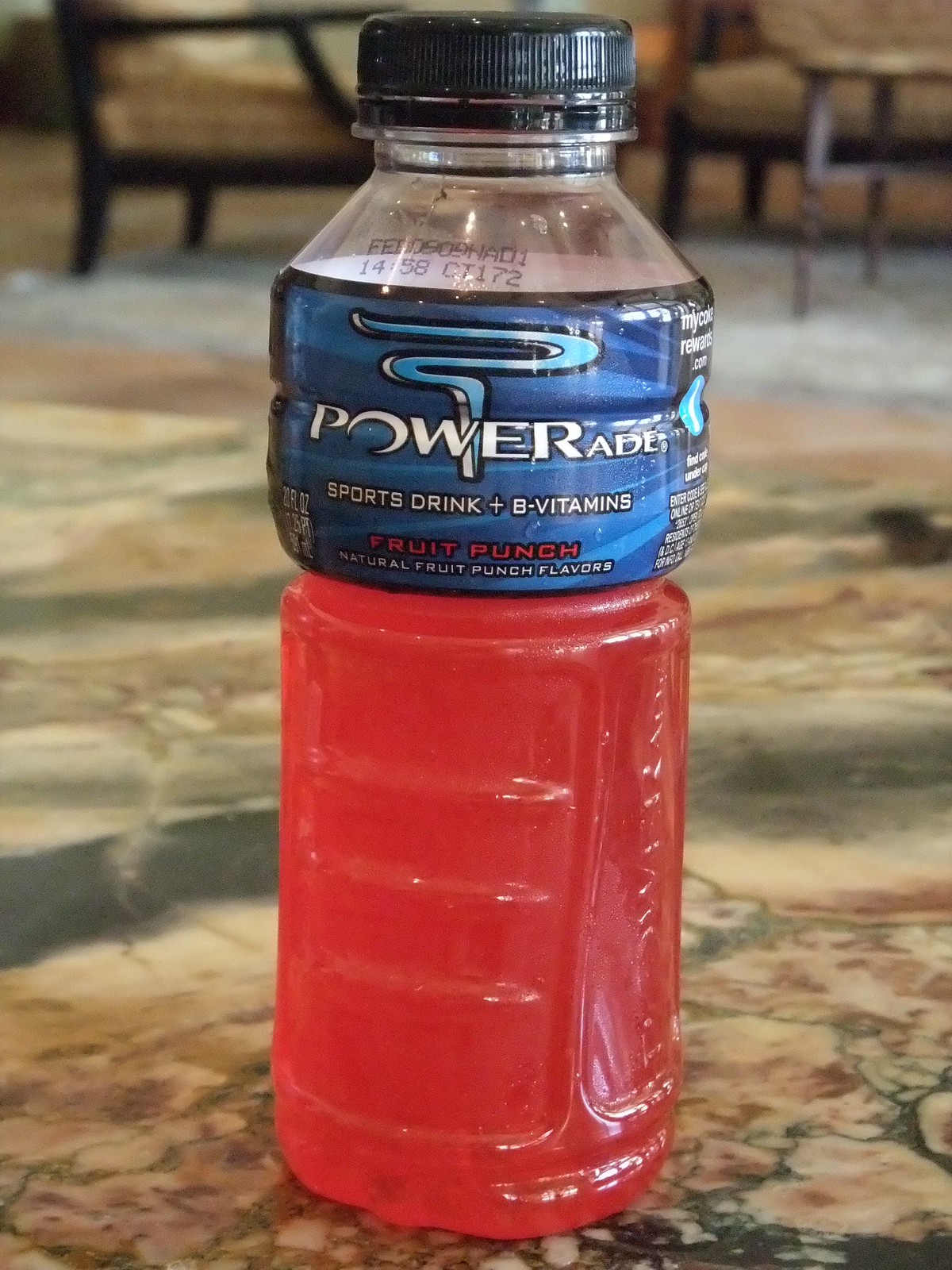This is a close-up photograph of a bottle of Powerade, specifically featuring the Fruit Punch flavor. The bottle's blue label prominently displays the Powerade logo and includes text that reads "Sports Drink + B Vitamins" and "Fruit Punch, Natural Fruit Punch Flavors." The label itself is predominantly blue and black, with additional details regarding the beverage. The Fruit Punch drink inside is a striking and vibrant red, typical of this type of flavored sports drink. The bottle is capped with a black top, which has already been opened, indicating that approximately one-third to one-fourth of the drink has been consumed, although the exact level is obscured by the label. The bottle rests on a mottled marble floor with hues of tan, orange, green, and light brown. The background is intentionally out of focus, but one can discern the presence of some low chairs, adding context to the scene without detracting from the central subject.